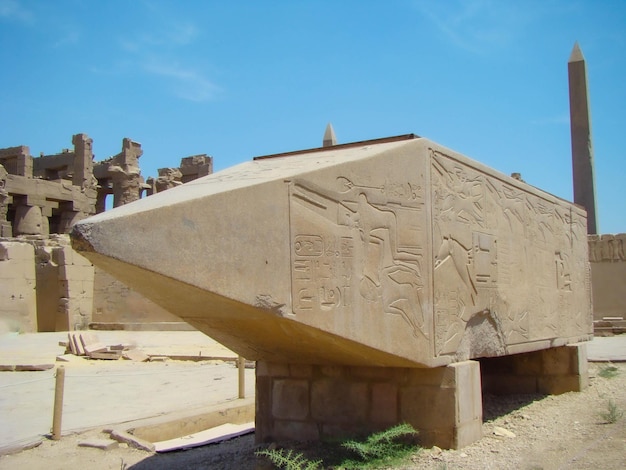This vivid colored photograph captures an outdoor scene featuring Egyptian ruins, with a clear blue sky overhead. The focal point is a large, tan obelisk, richly adorned with hieroglyphics, lying on its side and pointing from right to left. Its pyramidal top is clearly visible, while its base shows signs of damage. The obelisk is supported off the sandy, rocky ground by two substantial rectangular brick columns. In the background stands a taller, squared column with a pyramidal top, resembling the Washington Monument but distinctively Egyptian. Sparse patches of greenery, mainly a few small ferns, pepper the scene, especially around the fallen obelisk. This composition gives an impression of authenticity, enhanced by the presence of additional ruins in the background.